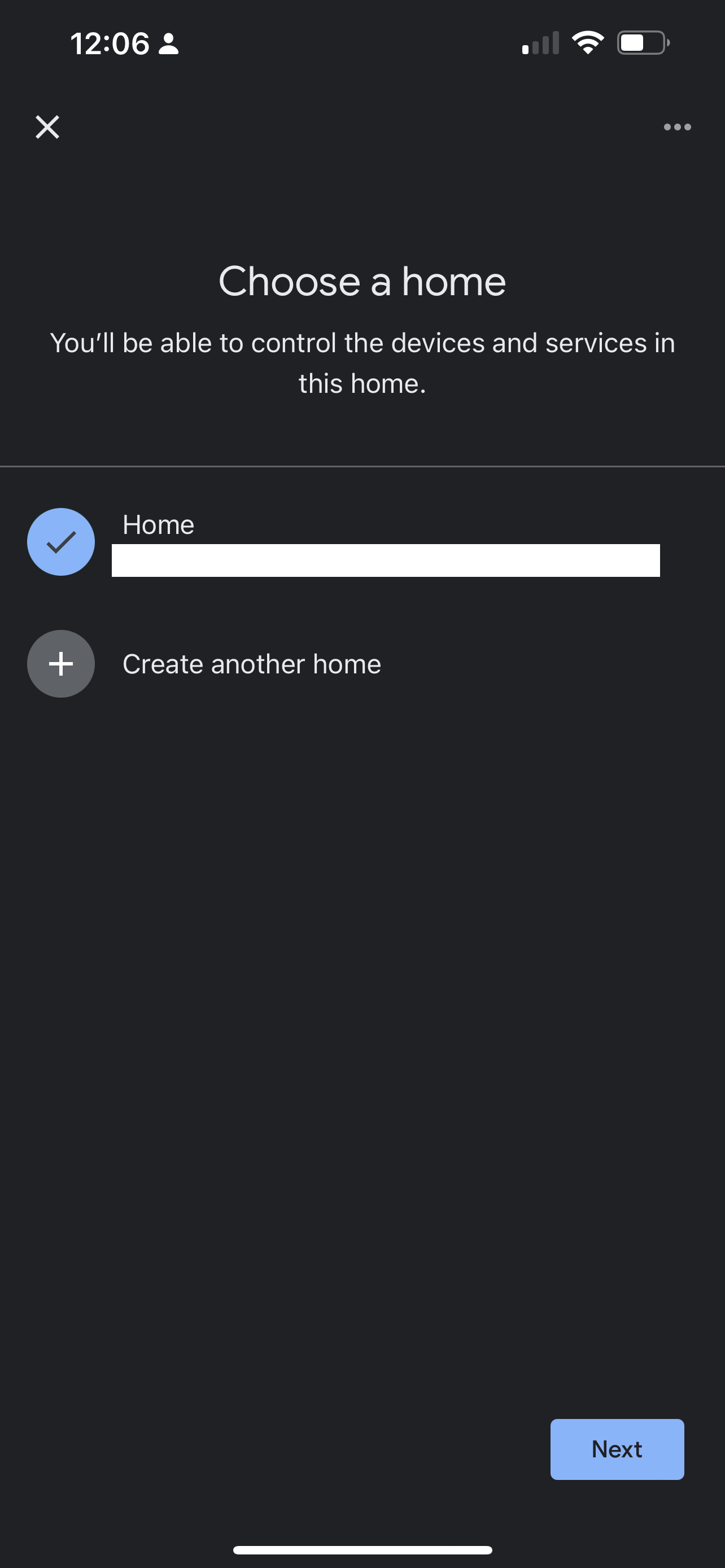Screenshot of a cell phone interface with a predominantly black background. The top part of the screen displays the status bar which includes the time "12:06", a small outline of a person icon, one active cell phone signal bar, full Wi-Fi signal, and approximately 50% battery life. Below the status bar, on the left-hand side, there is an "X" icon and on the right-hand side, there are three vertical dots suggesting a menu.

Centered in the screen is a message which reads: "Choose a home. You'll be able to control the devices and services in this home." Below this message, a horizontal gray bar spans from the left to the right sides of the screen.

Under the gray bar, a blue circle with a black check mark inside is displayed next to the word "Home" in white text. Beside this, there is an empty or possibly whited-out space, followed by a gray circle with a white plus sign inside. To the right of this circle, white text reads: "Create another home."

At the bottom right-hand side of the screen, there is a small grayish-blue button labeled "Next" in darker blue text. A slim white line is situated at the very bottom of the screen, completing the view of the interface.

There are no additional elements on this screen, and the description concludes here.